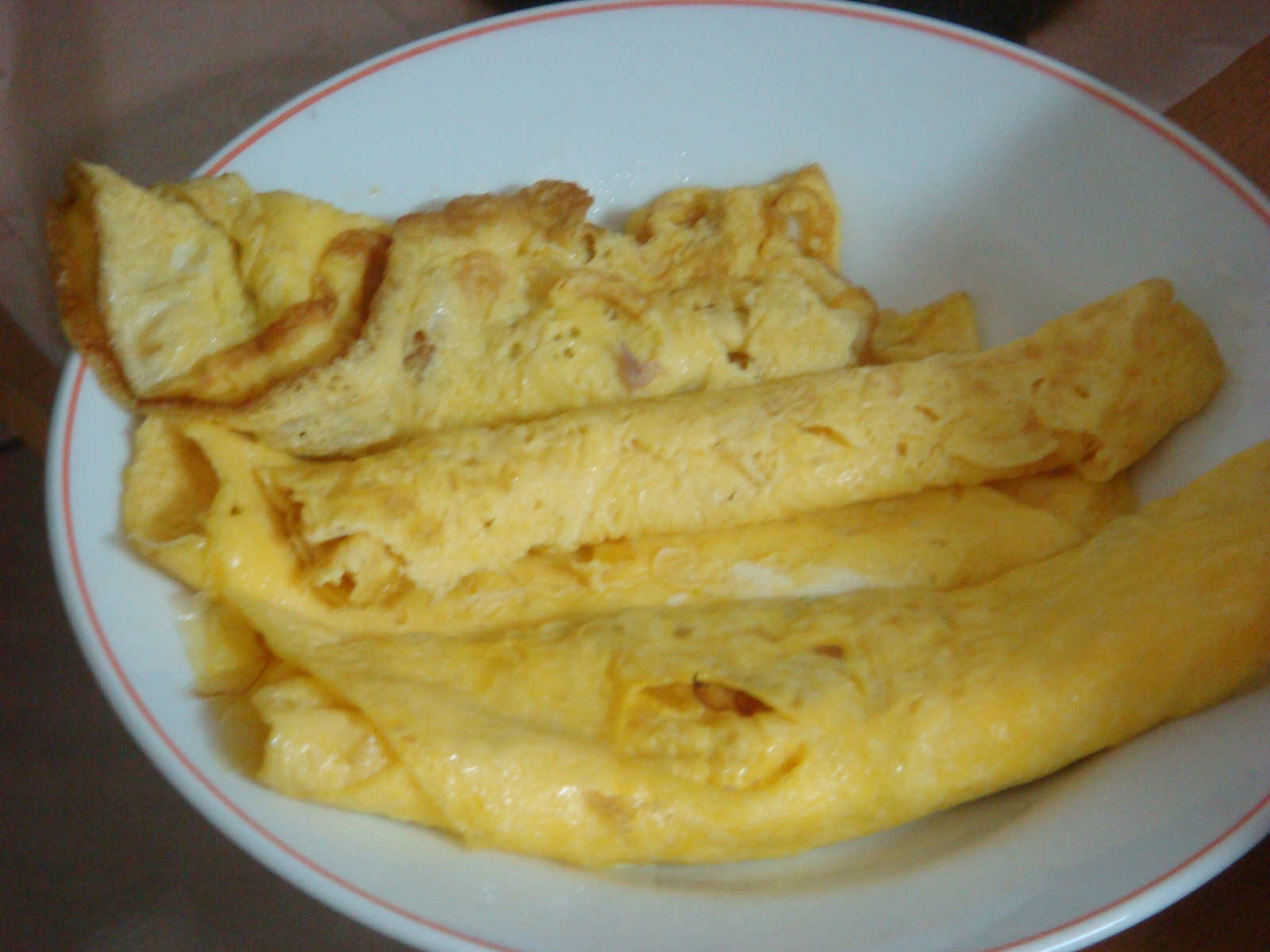In the photograph, a white porcelain plate, which slightly resembles a shallow bowl with a thin red or pink band around its edge, holds four rolled omelettes arranged horizontally across the plate. The omelettes appear thin, akin to crepes or taquitos, and are folded over, possibly encasing something simple like cheese, though it is unclear. The top omelette exhibits browned, crispy edges and contains pieces of ham poking through its surface, while the one at the bottom looks slightly undercooked and also shows hints of ham. The background is indistinct and grayish, suggesting the photo was taken under poor lighting and with low quality.